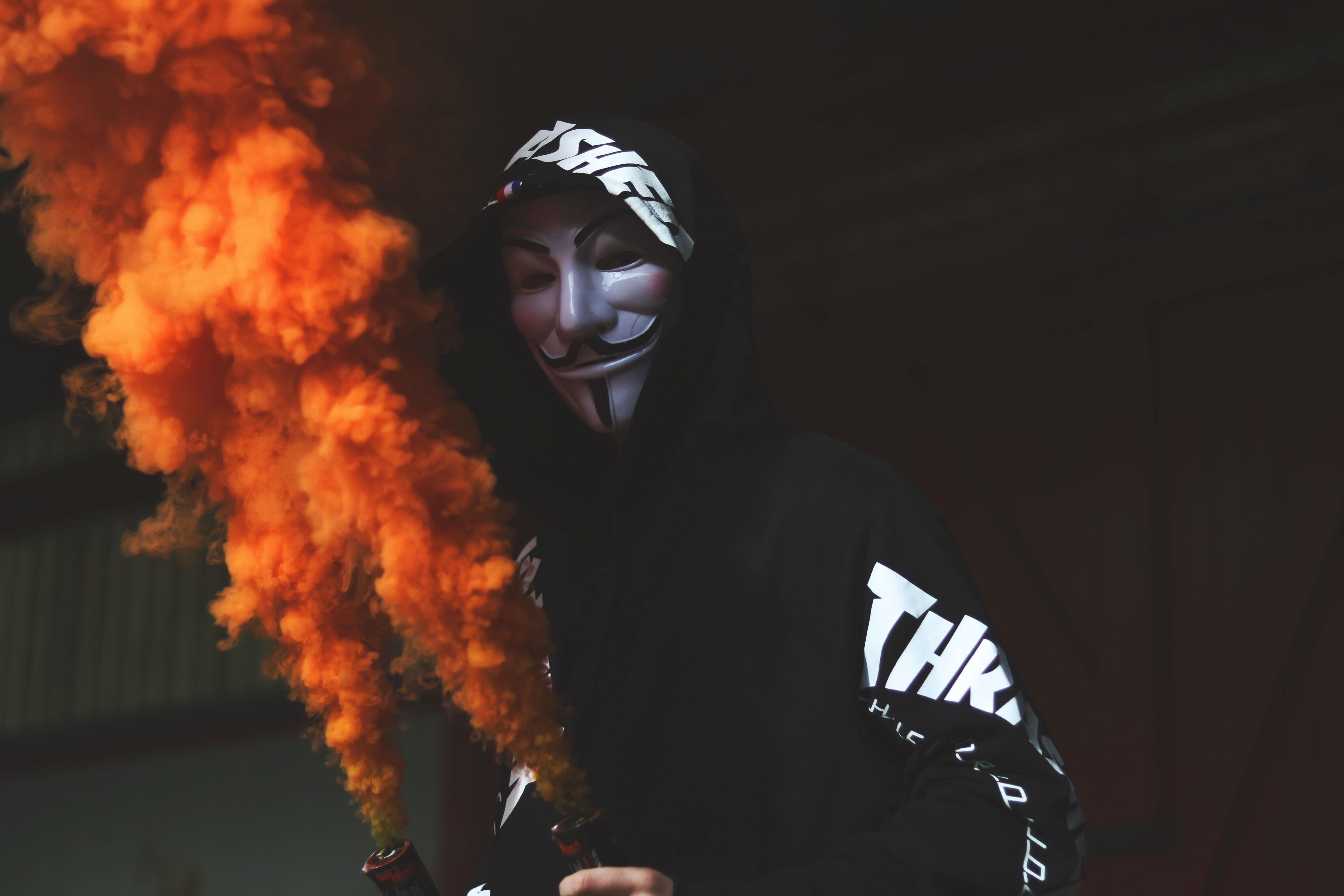The image depicts a human figure donning a white mask, reminiscent of the iconic Guy Fawkes mask. The mask features distinct attributes: a curved mustache beneath the white nose, a thin goatee under the mouth, and a long mouth line. The cheeks are adorned with large, rosy pink dots, and inquisitive, angled eyebrows are drawn above the eyes, adding to the mask's expressive demeanor. The figure is cloaked in a dark hooded sweatshirt, with the hood pulled up over their head. Visible on the hood are partially legible letters, spelling out "A S H E" and an additional letter that is obscured by the angle of the camera. The elbow of the sweatshirt appears to bear the word "THRASHER," although it is partially hidden. Underneath, more white lettering is present but obscured by a billowing cloud of orange smoke emanating from two cylinders held by the figure - one visible, while the other is partially cropped out of the frame. The overall ambiance is menacing, with a dark, indistinct background that might hint at a structure or setting but remains unclear due to lack of detail. The smoke and the figure's pose contribute to an ominous and dramatic scene.